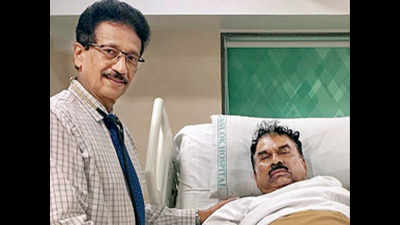In this photograph, there is a humorous and somewhat cinematic scene set in a hospital. A doctor, standing to the left, is looking directly at the camera with a smile on his face. The doctor is an Indian man with black hair and a mustache, wearing a checkered white and light brown plaid shirt, a loosely tied blue tie, glasses, and a stethoscope around his neck. His left hand rests gently on the shoulder of a patient lying in a hospital bed.

The patient, also an Indian man, appears to be in poor health, lying back with his head propped up on a light blue pillow. He has dark curly, messy hair, a mustache, and his eyes are closed, presenting a frowning, sickly demeanor. He is covered by a white sheet and a brown blanket pulled up under his arms.

The backdrop consists of a beige wall with a window on the right side, its green shade drawn down. The hospital bed, which is electrically adjustable, has noticeable side rails. The overall scene exudes a mix of authenticity and humor, largely due to the stark contrast between the smiling doctor and the dour patient.